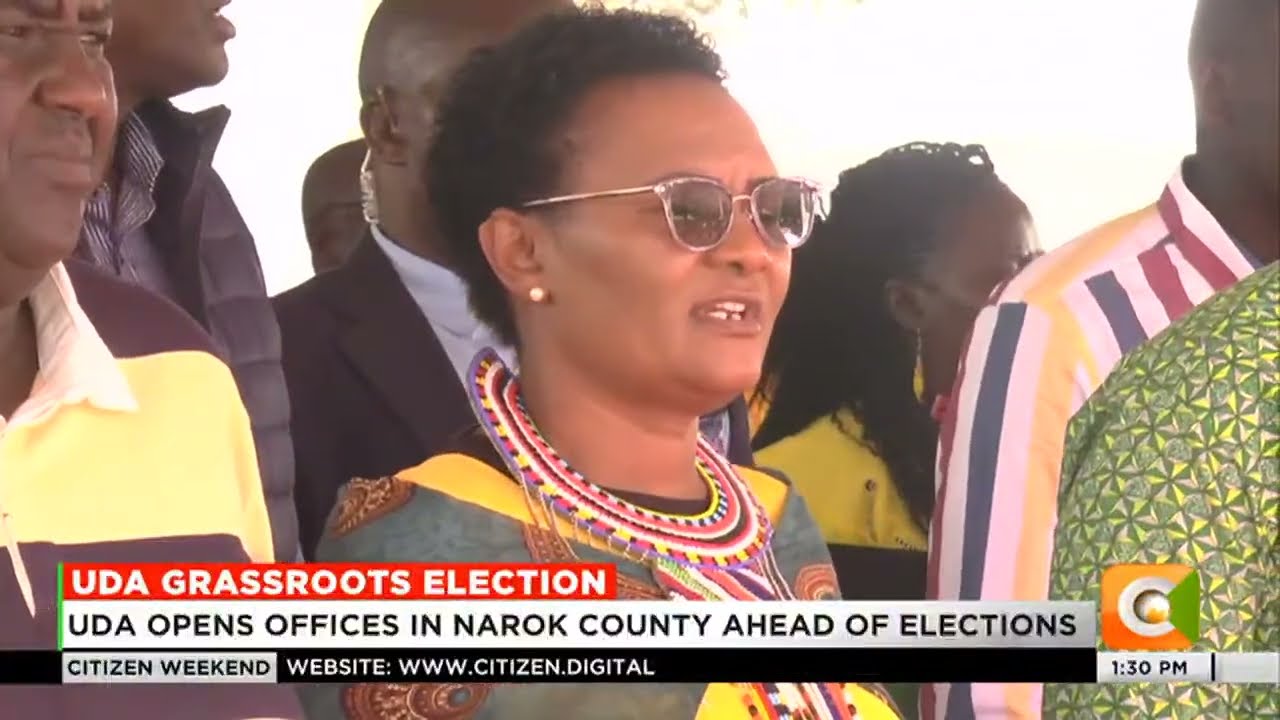The image, captured from a television news channel, features a diverse group of Black individuals standing together, presented in semi-formal attire. Prominently centered is a woman of African descent adorned with a distinctive beaded traditional neckpiece that cascades down her chest. She has short curly hair, is wearing tinted glasses, and a white pearl earring. Surrounding her are several men and women, slightly out of focus, suggesting a communal or formal gathering. Overlaid at the bottom of the screen is a series of horizontal bars providing news information in various colors: a red banner with white text reading "UDA Grassroots Election," a white banner with black text stating "UDA Opens Offices in Narok County Ahead of Elections," followed by "Citizen Weekend" and the website "www.citizen.digital." An orange square logo with a white circle and green hexagon is also visible, accompanied by a timestamp marking 1:30 p.m.